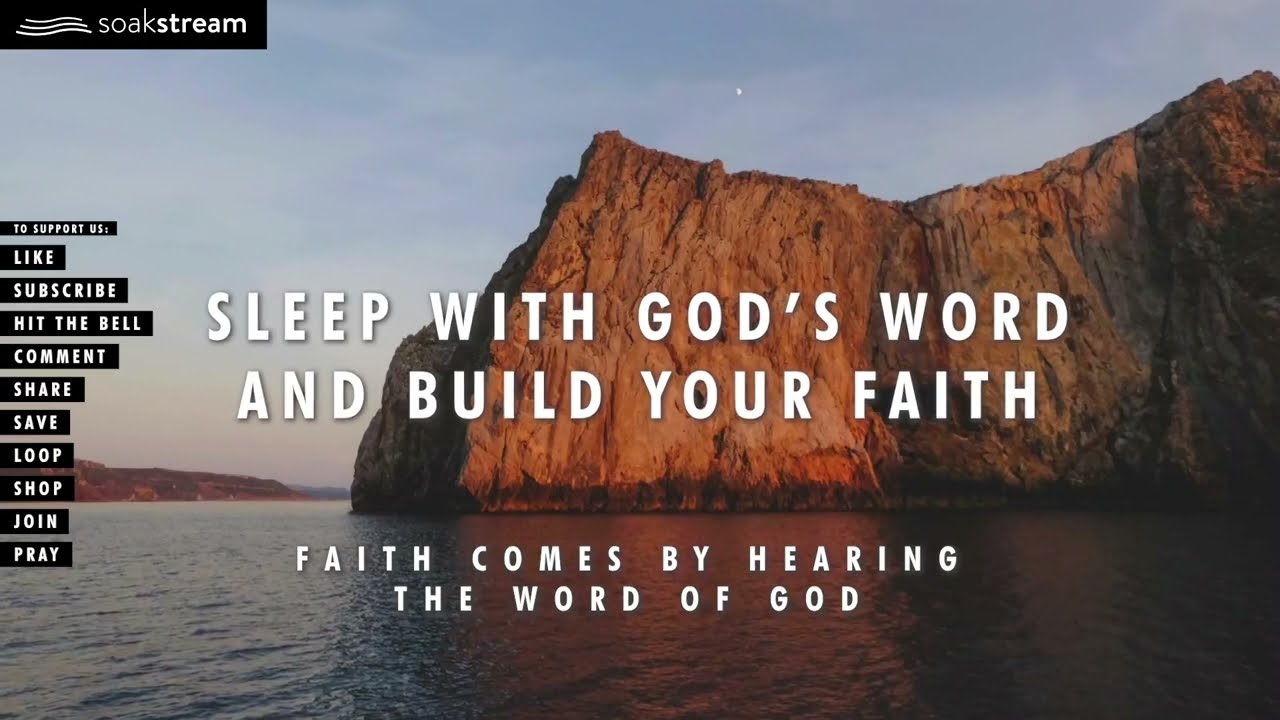The image appears to be a horizontally rectangular segment from a website or mobile app landing page designed with faith-based content. The foreground features prominent white, all-caps text centered across the middle that reads, "SLEEP WITH GOD'S WORD AND BUILD YOUR FAITH" followed by, "FAITH COMES BY HEARING THE WORD OF GOD." These lines are emphasized with a serene backdrop depicting a large rocky cliff emerging from a calm ocean, set against a dusky or dawn sky with thin marine clouds and a potential view of Jupiter. The top left corner displays the logo "SoakStream," with "Stream" bolded, accompanied by three wave-like shapes in white. Adjacent to the text, a black rectangular section lists navigational prompts such as "LIKE, SUBSCRIBE, HIT THE BELL, COMMENT, SHARE, SAVE, LOOP, SHOP, JOIN, PRAY," all in white, all-caps lettering, suggesting interactive elements typical of a YouTube thumbnail.